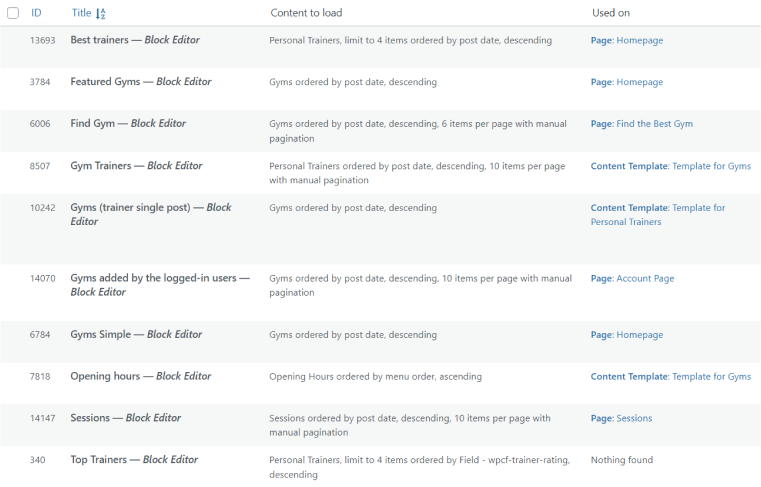This image showcases a detailed itemized list with alternating gray and white backgrounds for each entry. At the top, there is a header that features a checkable box along with the following labeled columns: "ID," "Title," which is sortable in ascending (A to Z) and descending order, "Content to Load," and "Used On."

### Detailed Breakdown of Items:
1. **ID Number:** 13693
   - **Title:** Best Trainers - Block Edition
   - **Content to Load:** Personal Trainers
   - **Order:** Limited forward items ordered by post date (descending)
   - **Used On:** Home Page

2. **ID Number:** 3784
   - **Title:** Featured Gyms - Block Editor
   - **Content to Load:** Gyms
   - **Order:** Ordered by post date (descending)
   - **Used On:** Home Page

3. **ID Number:** 606
   - **Title:** Find Gym - Block Editor
   - **Content to Load:** Gyms
   - **Order:** Ordered by post date (descending), six per page with manual pagination
   - **Used On:** Find the Best Gym Page

4. **ID Number:** 8507
   - **Title:** Gym Trainers - Block Editor

Each entry on this list methodically details relevant information like the identifier number, title, type of content, sorting order, and the specific page it is used on. This organized layout ensures easy navigation and understanding of the listed items.